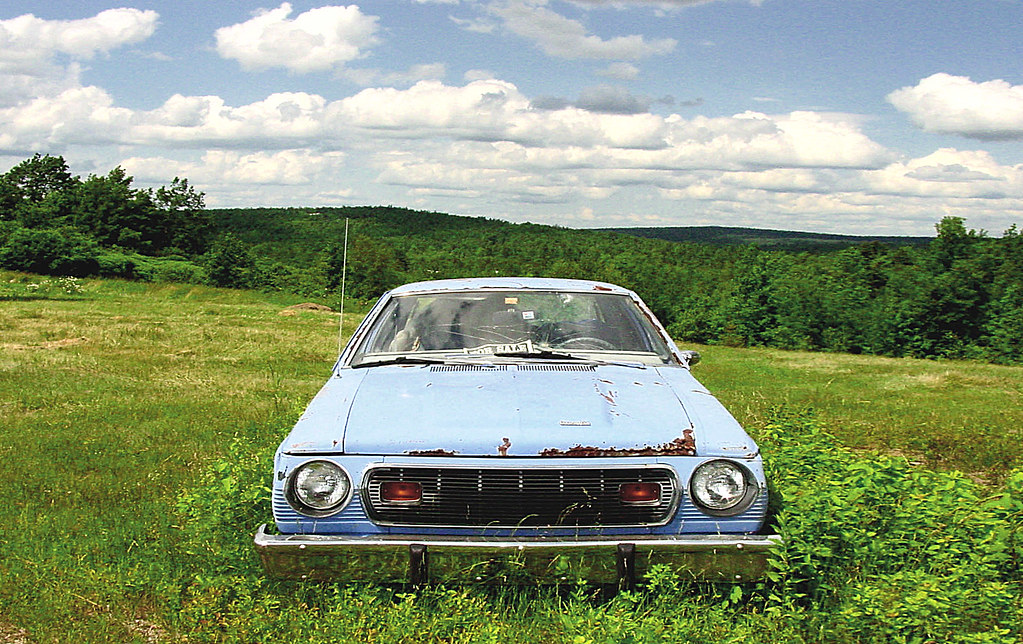The photograph captures a serene outdoor scene during the daytime, dominated by a sky filled with wispy white clouds and a clear patch of blue in the top right corner. Front and center in the image is an old, baby blue car that appears to have been abandoned in a lush, green field for a significant amount of time. The car is an older model, showing signs of age with rust on the hood and a cracked windshield, yet it remains in relatively decent condition with its chrome bumper still shiny enough to reflect the surrounding vegetation. Around the car, weeds are growing, particularly near its bumper, while the grass in the background is shorter. Behind the car stretches an expanse of green trees and hills, creating a scenic, natural backdrop that extends to the horizon. The focus of the image is unequivocally on the car, positioned centrally and facing the viewer, standing alone amidst the lush greenery.